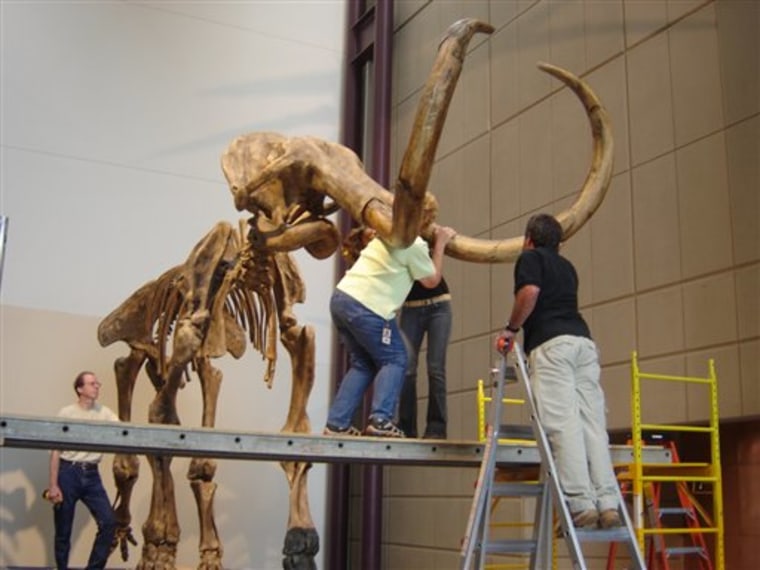In this detailed image, a team of four individuals is meticulously assembling the skeletal structure of a colossal woolly mammoth or a similar elephantine creature. The focal point of their effort is the creature's massive tusks, which appear enormously impressive against the skeletal frame. The majority of the team is utilizing metal scaffolding and ladders, ensuring they can reach and position the tusks correctly. At the front, two people are diligently working together to secure the tusks, while a third person on a stepladder appears to be aiding in the process or overseeing the alignment. In the background, a man dressed in jeans and a white shirt stands where the mammoth's tail would be, observing the progress and possibly supervising. The scene is set within a spacious museum or large building, identifiable by its high ceilings and a beige-paneled wall with geometric designs on the right. The dark coloration of the bones suggests they are ancient, adding historical weight to the scene. The image is taken from a 45-degree angle, providing a comprehensive view of the assembly process and the grand scale of the exhibit.